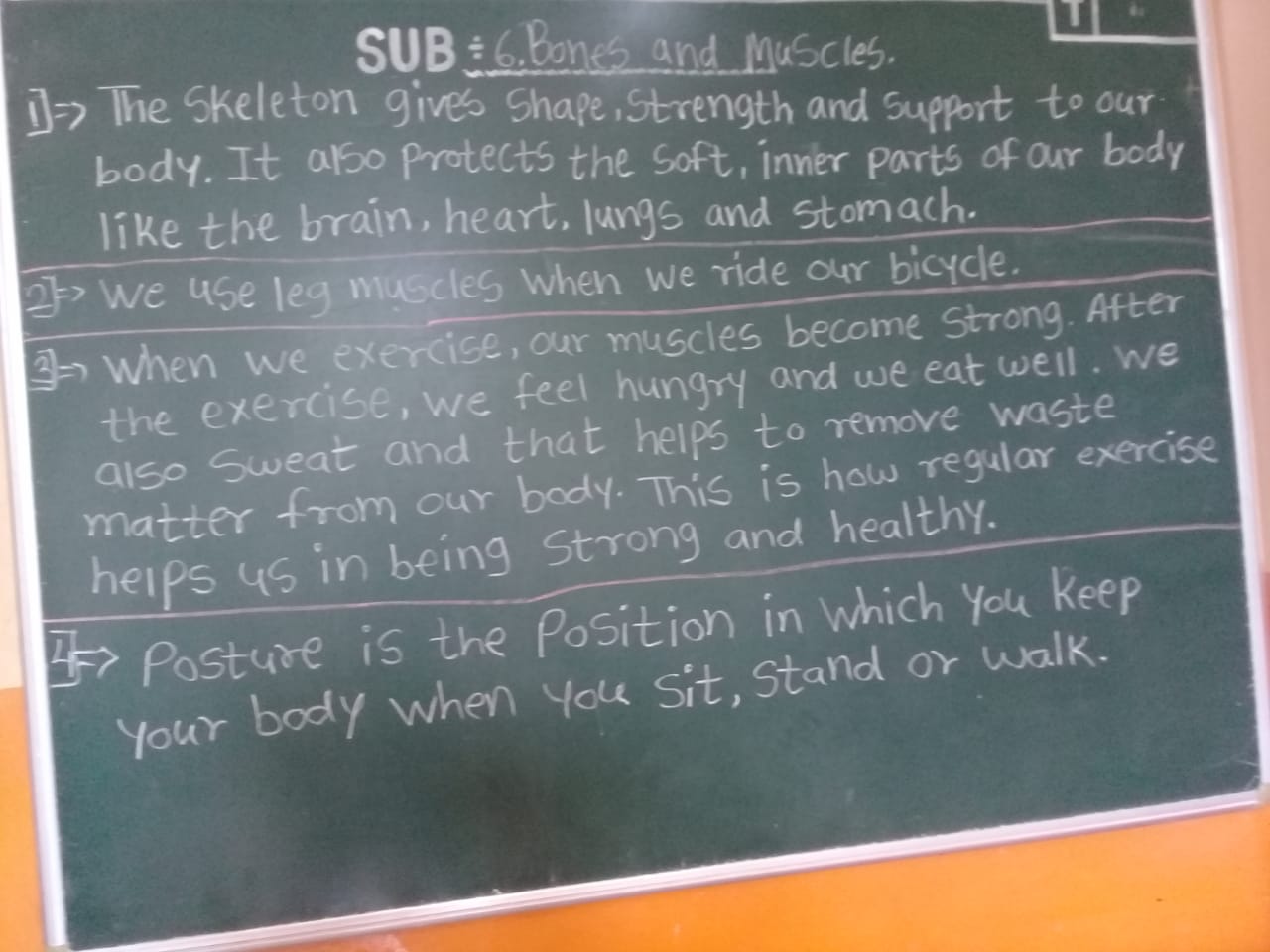The image appears to be from a school in a developing country, possibly in Africa. The classroom is modestly equipped, lacking modern amenities such as a whiteboard or projector. The focus of the lesson is on human anatomy, specifically teaching bones and muscles to what seems to be middle school-aged students. The chalkboard displays the subject matter clearly, with a heading that reads "Bones and Muscles," alongside a brief description stating that the skeleton provides strength, shape, and support to our bodies. The educational setting is indicative of a dedicated effort to teach fundamental health and biology topics despite limited resources.